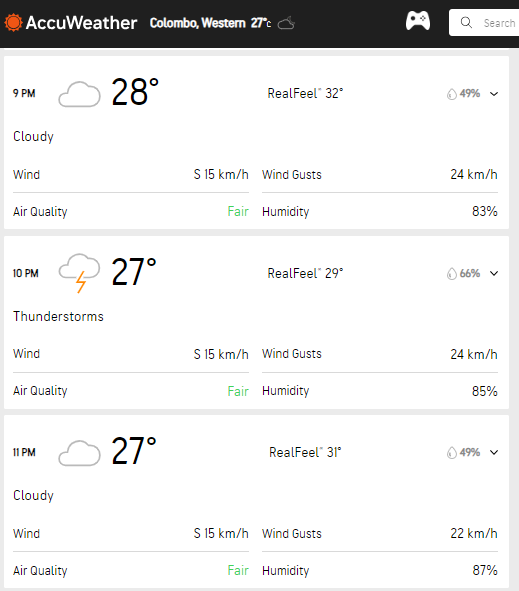The screenshot in consideration is from AccuWeather, featuring a search bar and a gaming icon. It displays weather conditions for Colombo, Western, with a current temperature of 27°C. The detailed hourly weather forecast is as follows:

- **9:00 PM**: The temperature is 38°C, with a "RealFeel" of 32°C. Humidity stands at 49%, and the sky is cloudy. Wind speeds are 15 kilometers per hour with gusts reaching 24 mph.
  
- **10:00 PM**: Thunderstorms are expected, with a "RealFeel" of 29°C. The humidity rises to 66%, accompanied by winds at 15 mph and gusts up to 24 mph. The air quality is fair, and overall humidity is at 85%.

- **11:00 PM**: The temperature drops to 27°C, with a "RealFeel" of 31°C. Humidity increases to 87%, and the air quality remains fair. Wind gusts reduce to 22 mph, and it's forecasted to be cloudy, with winds at 15 kilometers per hour.